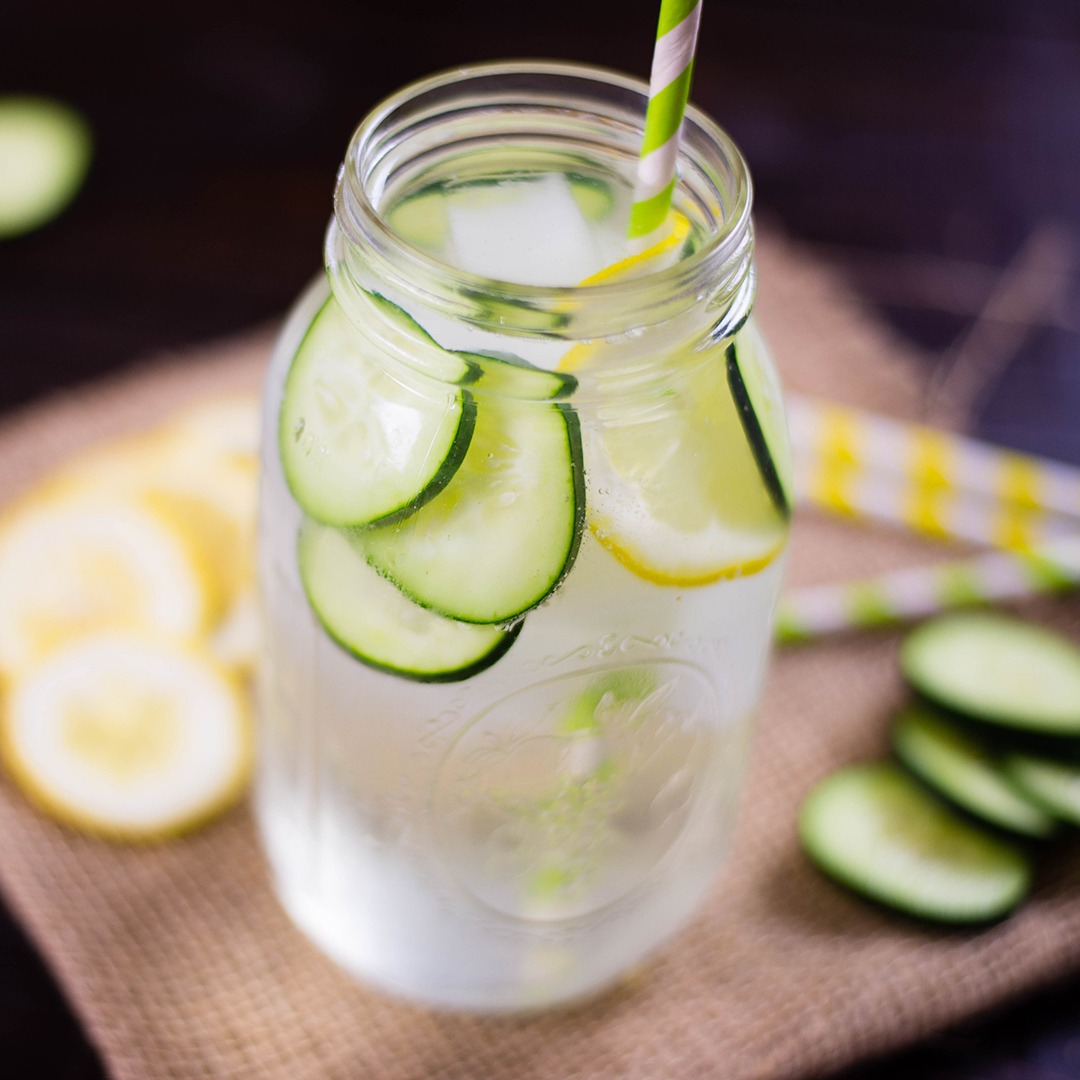This square photograph vividly captures a refreshing beverage in a clear mason jar, which is positioned as the central focus of the image. The drink appears to be a clear, ice-filled lemonade, adorned with floating slices of cucumber and lemon. Emerging from the jar is a lime green and white striped straw. Surrounding the jar is a burlap fabric placemat that enhances the rustic aesthetic, dotted with scattered lemon and cucumber slices, as well as additional yellow and white striped straws. The background is dark and intentionally blurred, directing all attention to the inviting, well-composed drink that sits ready to be enjoyed.